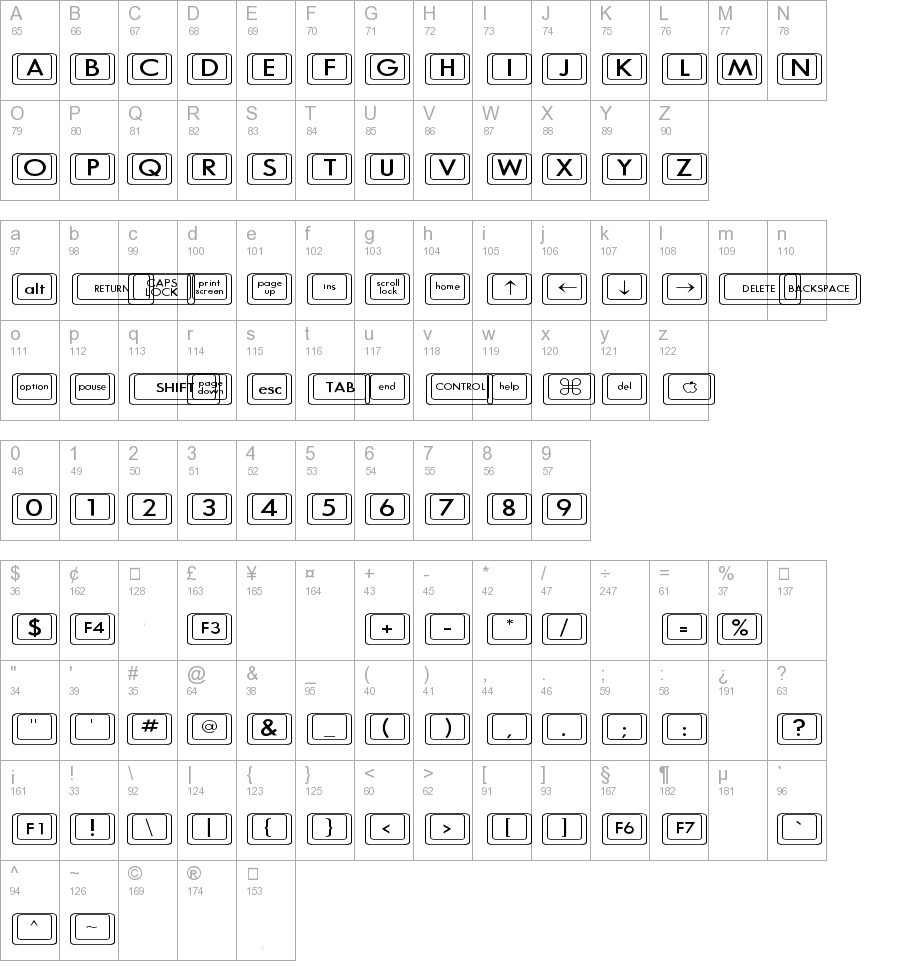This image showcases an extensive and detailed visual representation of a keyboard. At the top, there's a sequence of uppercase alphabetic keys starting with 'A' and continuing to 'Z', each displayed in a standard light gray font. Alongside each letter, a corresponding number is indicated, beginning with 65 for 'A' and incrementing sequentially to 90 for 'Z'. Below this row of upper-case letters, smaller case letters are presented, paired with a variety of essential keyboard function keys. These include 'Alt', 'Return', 'Caps Lock', 'Print Screen', 'Page Up', various arrow keys, 'Delete', 'Backspace', 'Shift', 'Tab', and 'Control'. Additionally, a row of digit keys from 0 to 9 is featured, followed by keys from the number pad. The image also depicts special characters and function keys, such as the hashtag (#), ampersand (&), F1 key, exclamation point (!), question mark (?), and various other punctuation marks.